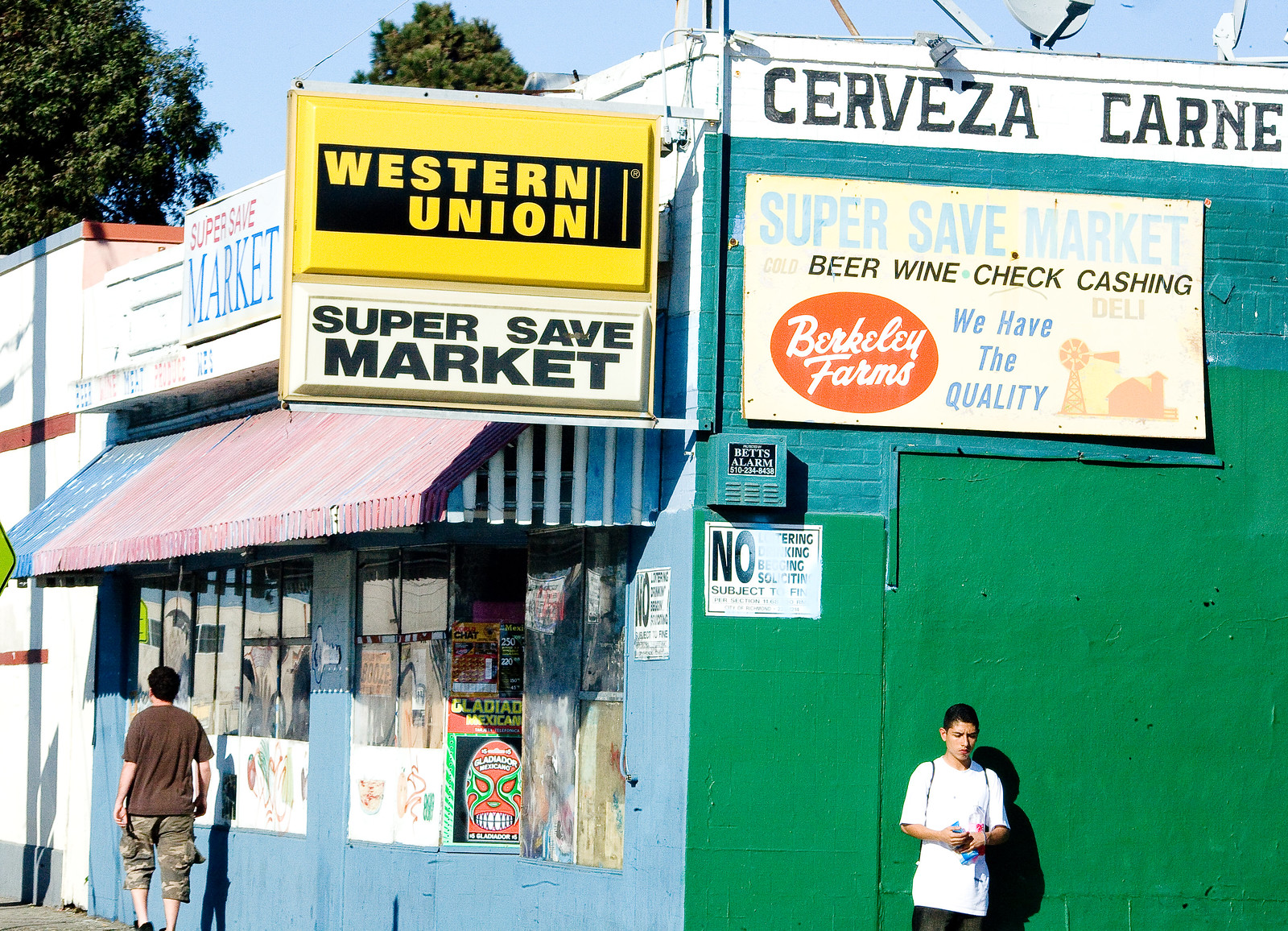The photograph captures the exterior of a small, old-fashioned corner market under a bright, cloudless sky. The market, identified as "Super Save Mart," has a storefront marked by a combination of teal and green bricks that transition into smooth cement at the lower sections. Prominently displayed at the front and side of the building are multiple signs. At the top center-left, a bright yellow "Western Union" sign with a black border can be seen. Directly beneath it, a rectangular sign announces "Super Save Mart" in black text on a white background.

Above the storefront, on a white background, the words "Cerveza Carne" are visible in black lettering. Another large sign below reads "Super Save Mart Beer Wine Check Cashing," featuring a red oval with "Berkeley Farms" and an image of a farm with a barn and windmill, accompanied by the text "We Have Quality."

The front of the market is adorned with a plethora of signs and posters on the windows, and a prominent awning designed to resemble the American flag—blue with white stars on the left side and vertical red and white stripes in the center—provides shade to the entrance. 

In the scene, a teenager with tan skin, dark black hair, and wearing a white T-shirt and backpack straps is located near the bottom right of the image, leaning against the side of the market. Another pedestrian, dressed in a brown shirt and camouflage cargo shorts, walks past the front of the market with his back turned to the camera. In the background, green trees and a clear, light blue skyline frame the bustling market scene.